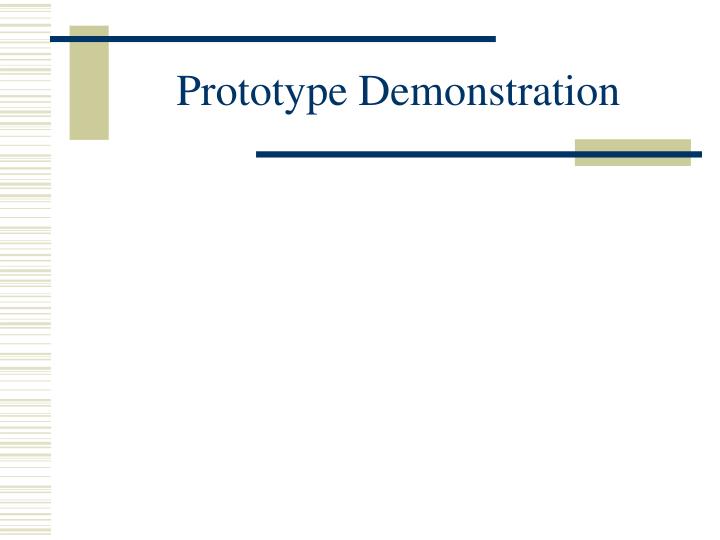The graphic is a minimalist PowerPoint slide template with a predominantly white background. Along the far left, a vertical stripe composed of variously sized beige and gray horizontal lines creates a barcode-like design. This distinctive design element anchors the left side of the slide and is paired with a smaller beige line at the top left corner. The centerpiece of the slide features dark blue text stating "Prototype Demonstration," flanked above and below by thin blue horizontal lines. The top blue line is intersected by a vertical beige bar, and there is another small beige rectangle aligned with the bottom blue line. The overall layout is simple and clean, making it an ideal template for adding more text or images, possibly for a prototype demonstration presentation.